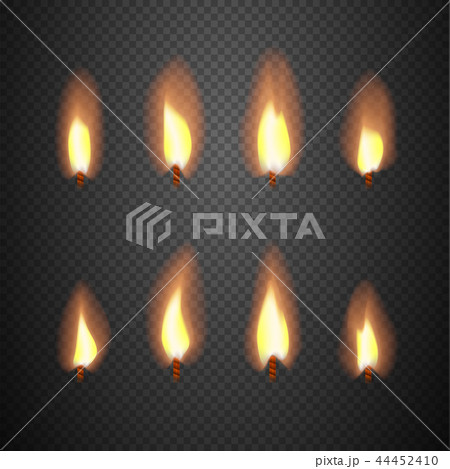In the image, a gray and black checkerboard background frames the scene, with very small checkers creating a textured effect. Dominating the image are eight upright candles arranged in two rows of four, each topped with a lit flame. These flames exhibit varied shapes, lengths, and widths, displaying a core of yellow and white with an orange-red glow encircling each. Notably, the flames are distinct, each with a unique red-orange halo differing from the others. Centered and slightly to the left, a triangular or diamond-shaped emblem features the text "PIXTA," with additional text below reading "PIXTA JP 444-52410." A subtle, incomplete X made of light gray lines crosses through the middle, indicative of a watermark typical of stock imagery. The overall style has an animated aesthetic rather than a realistic one. The image includes colors such as orange, yellow, red, gray, black, and white.